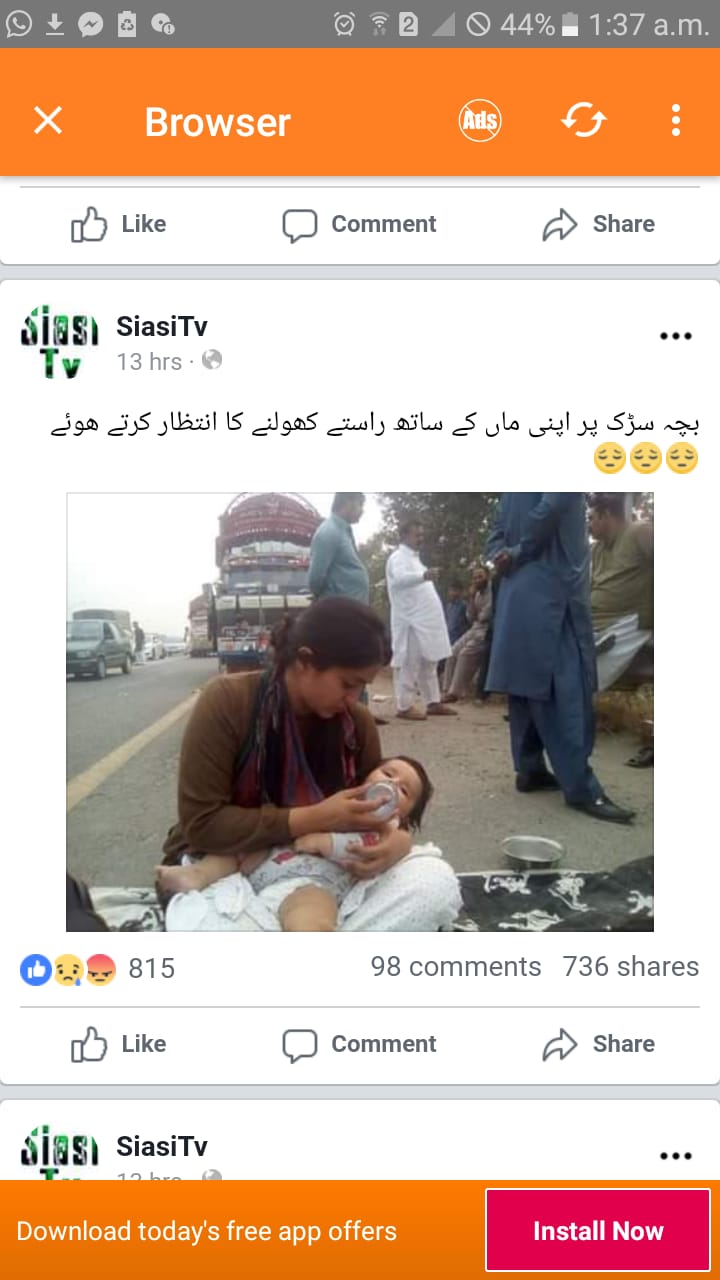The image is a color screenshot from a mobile phone, displaying a Facebook post. The screenshot features the typical smartphone interface elements, including a browser heading with an orange border, battery power, signal strength, and time indicators at the top. The post is from a page called Siasi TV (S-I-A-S-I TV) and is predominantly written in what appears to be Arabic or a language from the Middle Eastern/Indian subcontinent.

Central to the image is a poignant photograph of a woman, who appears to be from the Middle East or South Asia based on her clothing and surroundings. She is sitting on a mat, holding a baby in her arms and feeding it with a bottle. The scene is set on a busy street, surrounded by vehicles and onlookers, mostly men dressed in traditional garments from that region.

Above the photograph, there are social media reaction icons, including thumbs up, sad, and angry emojis. The post has garnered significant interaction, with 815 reactions, 98 comments, and 736 shares. At the bottom of the image, there are interactive buttons for liking, commenting, and sharing the post. Additionally, there's a promotional banner with a red button suggesting downloading an app.

In summary, this detailed screenshot captures a moving moment of a woman feeding her baby amidst a busy street, highlighting social media's power to evoke strong emotional responses and widespread engagement.